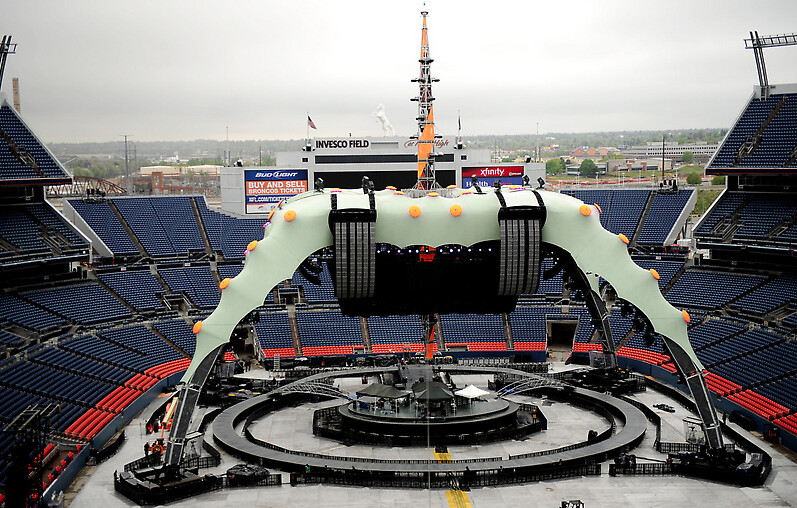The image captures a high-angle view of Invesco Field, the stadium renowned as the home of the Denver Broncos. In the background, atop the scoreboard, the stadium’s name "Invesco Field" is prominently displayed alongside a horse, confirming its association with the Broncos. Advertisements for Bud Light, Xfinity, Buy and Sell, Broncos Tickets, and NFL.com/tickets also adorn the scoreboard. The stadium’s stands are visible, showcasing a sea of blue and orange seats, juxtaposed against the backdrop of the cityscape, which includes homes, trees, and a partly cloudy sky providing ample natural light.

At the center of the stadium, a large setup suggests preparations for an upcoming event, likely a concert. The stage, a circular structure with an inner circle connected to an outer circle, features black and white tents within it. An imposing orange tower rises from the structure, flanked by vertical lines of lights that reinforce the stage’s dramatic presence. The unique design of the stage, with its overhanging elements that almost resemble the limbs of an octopus adorned with button-like features, adds a futuristic touch to the scene.